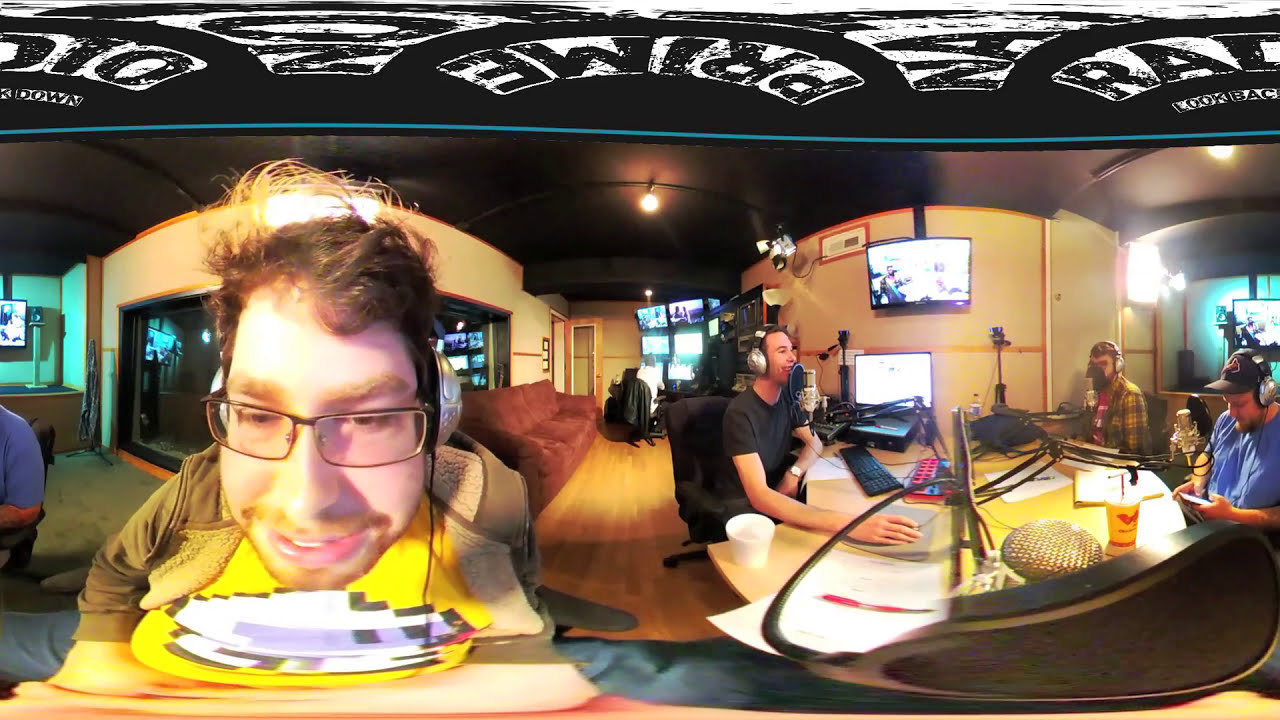The image is a 360-degree panoramic view of a high-end recording studio, possibly used for a podcast, radio show, or talk show. The room features brown walls and a brown wood floor, with a red couch and multiple TV and computer monitors arranged around the space. At the center of the scene is a round table where four men are seated, each equipped with a microphone and wearing headphones. There are also keyboards, a mouse, and a laptop on the table, suggesting an interactive and technical setup. 

On the far left, there's a man in a blue shirt, partially captured with only his shoulder visible. Continuing to the right, we see the likely photographer, a white male with disheveled brown hair, wearing glasses and a brown shirt with a bright white and yellow logo. Further along, another man sits behind numerous monitors, possibly handling video production tasks. 

The main table hosts several participants: another man in a blue shirt looking down at his smartphone and a man in a plaid shirt, both wearing headphones and engaged in the conversation. The image, characterized by its fisheye distortion, shows a meticulously arranged studio with a well-lit, black ceiling and a lively atmosphere as everyone appears to be laughing and enjoying the discussion. The presence of multiple cameras and live feed displays on the wall underscores the professional and high-tech environment of this recording setup.